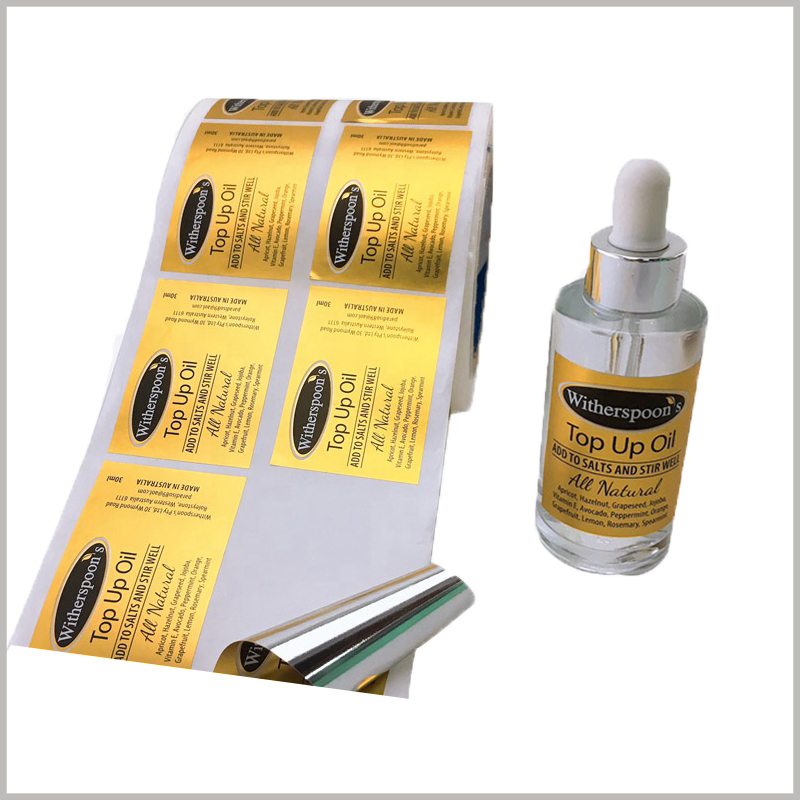The image depicts a roll of gold foil stickers set against a completely white background. The stickers, featuring black text within a black oval at the top, read "Witherspoon’s top up oil, add to salts and stir well, all natural," and list ingredients such as apricot, hazelnut, grape seed, vitamin E, avocado, peppermint, orange, grapefruit, lemon, rosemary, and spearmint. One sticker is being peeled off from the roll, revealing a silver backing. Adjacent to the roll is a clear container with a lid and an eyedropper, partially filled with clear liquid, which already has one of the stickers adhered to its front. These labels are intended for these bottles of oil, suggesting that the oil might be used for health purposes.